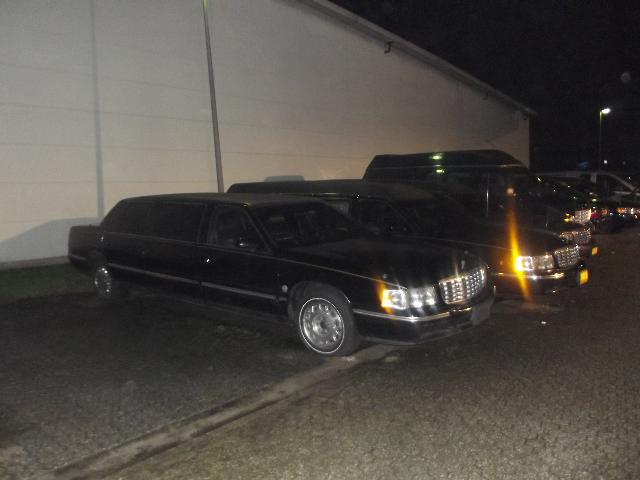This nighttime color photograph captures a scene featuring a row of dark-colored vehicles parked alongside a light-colored building with a sloping roof. The building, made of cinder blocks and painted off-white or light tan, has thin horizontal gray lines and a gutter hanging at the roof's edge. In the background, a black sky contrasts with the distant glow of a street light on the right-hand side. The foreground prominently displays two black limousines with chrome wheels and illuminated parking lights, casting a glare. The front limousine has its headlights on, and the reflection of its grill is visible. Next to the limousines, partially visible, is a large black van, followed by another dark-colored vehicle further in the distance, possibly a black SUV. The paved area in front of the building features a cobblestone road and a walkway with a geometric pattern, and additional cars can be seen trailing off into the background, though they are not clear enough to describe accurately.